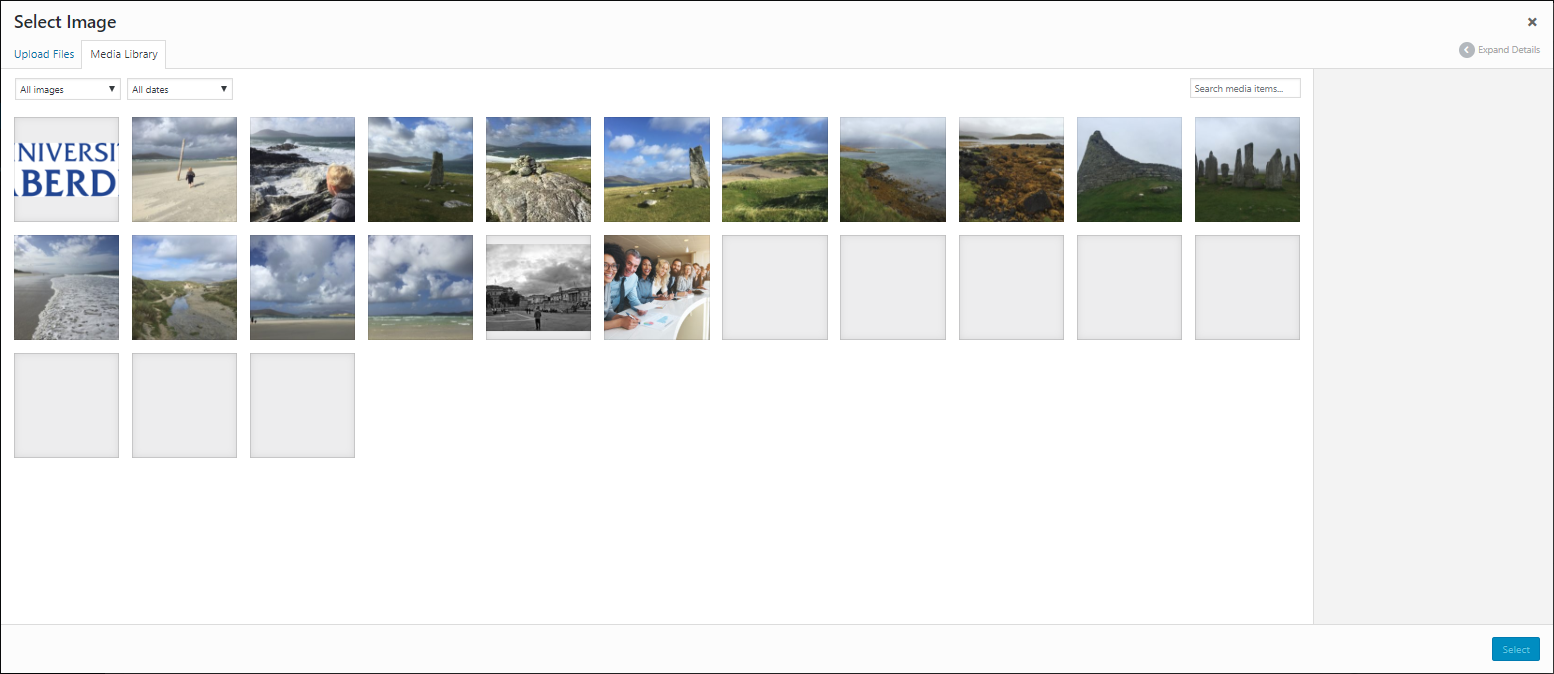This image showcases a computer's media library interface. At the top of the screen, the bold black text "Select Image" is prominently displayed. There are two clickable options: "Upload Files" in blue text and "Media Library" in black text, with the latter being the currently selected tab. 

The media library is filled with a grid of images across multiple rows. In the first row, there are eleven images. The second row also features eleven squares, though only six of them contain images, leaving five empty gray boxes. A third row has begun, with three additional gray boxes present.

Towards the top right of the interface, an X icon allows the user to close the window. Adjacent to this, a left-pointing arrow within a gray circle is labeled "Expand Details." At the bottom right corner of the screen, a blue "Select" button is clearly visible, enabling the user to choose an image for their needs.